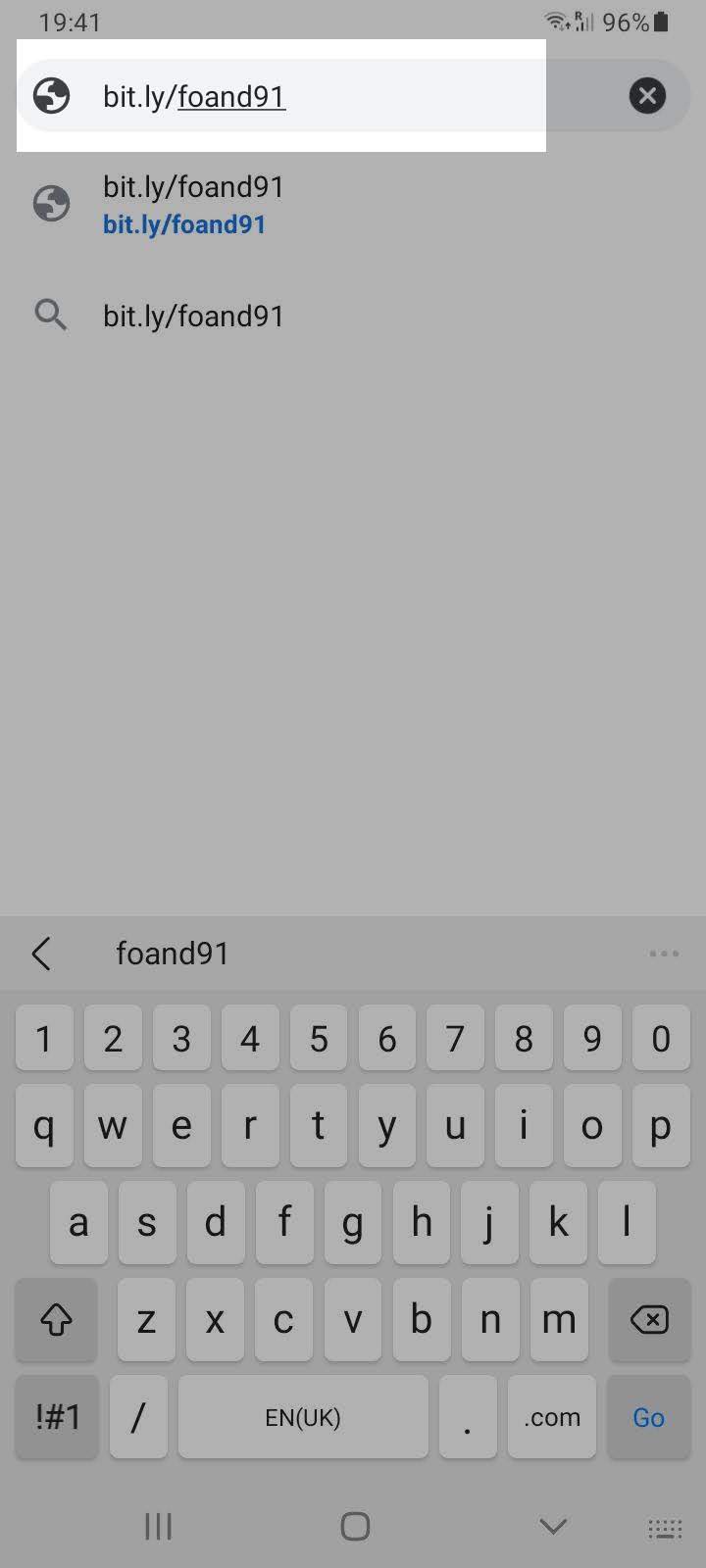**Detailed Caption:**

Featured in the image is a simplistic yet informative layout on a white background that transitions to a gray hue at the top, blending into a black gradient. The image appears to be from a user interface or electronic screen circa 1941, detailing various statuses and icons that include cell strength, Wi-Fi strength, cell strength, and a roaming indication, all alongside a 96% battery life highlighted in white.

A central element in the image is a URL visibly shown multiple times: **bit.ly/foN91**. The part 'foN' in the URL is underlined, drawing attention to it. To the right of this URL, there is a prominent black circle encompassing a blue 'X'.

Beneath this primary URL and its black circle with blue 'X', another version of the URL appears without underlining, followed by a third repetition of the link in blue text. Below this set, there is an icon resembling a magnifying glass in gray.

Towards the bottom of the image, a sequence of elements is displayed, starting with the URL repeated in black text. An arrow pointing to the right stands adjacent, succeeded by the typed entry of the URL yet again.

A quirky virtual keyboard dominates the lower section of the image, featuring white keys with black text. Keys include standard characters along with special symbols: an exclamation point, pound sign, and the numeral one. On the right side, the keyboard houses a delete button and a blue 'Go' button, indicating execution or submission.

The bottom section of the keyboard exhibits additional functionalities: a three-lined square suggesting menu access, an arrow (gray or 'V') pointing downward, and a newer keyboard symbol that appears to be less commonly used.

All these elements together convey an intricate representation typical of an interface laden with informational and interactive features, encapsulating a vintage, yet highly detailed snapshot.